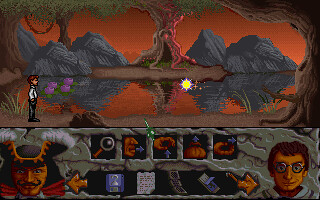This screen capture from a game console features a vibrant, predominantly orange background. Dominating the scenery are large, brown trees positioned on the left and right upper edges of the image, along with another tree centered at the top. These trees are adorned with green leaves that extend horizontally across the upper section, adding a splash of contrasting color. Below, a series of rocky hills stretch across the horizon, while in the center lies a tranquil, lake-like surface. The water appears orange, reflecting hints of purple and yellow, suggesting a surreal or fantastical setting. In the foreground, tall grass grows along the lake's edge, further enriching the landscape. A male character, dressed in a white shirt and black pants, stands at the center-left edge, gazing towards the right. Adding intrigue to the scene, two large head figures occupy the lower corners: the one on the left resembles a pirate, while the one on the right bears a striking resemblance to Harry Potter.